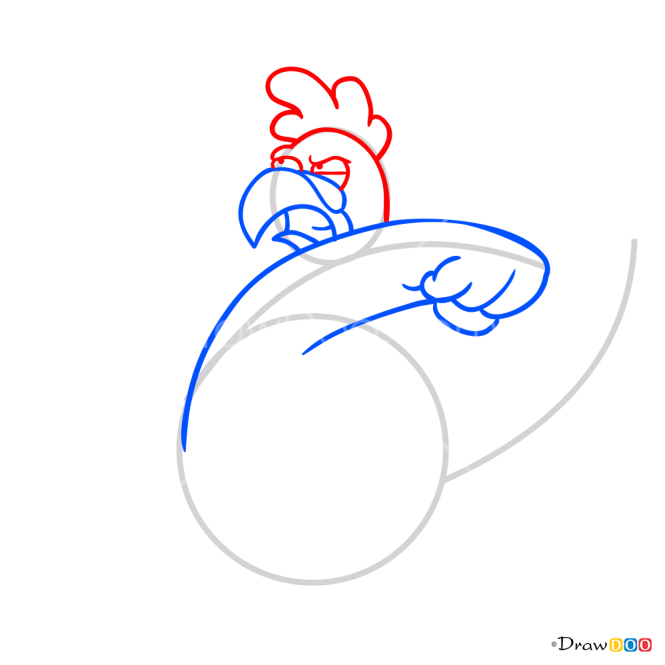In this digitally created image, the background is entirely white, enhancing the simplicity and focus on the central figure—a cartoon chicken depicted with an angry expression as it throws a punch. The chicken's design includes a white oval head with a blue beak, striking red eyes, and a red comb resembling a mohawk. The body is minimal, outlined by basic gray shapes, including a circle and a curved line that forms the punching arm, which is highlighted in blue.

At the bottom of the image, "draw 000" is written unobtrusively. Nearby, positioned neatly in the bottom right corner, is a small, non-intrusive company logo that incorporates colors such as yellow and black. These colors, along with white, red, blue, and gray, are consistent throughout the image. The overall style suggests that this could be used as a versatile company logo, suitable for use on the side of a truck, a business facade, or a company website.